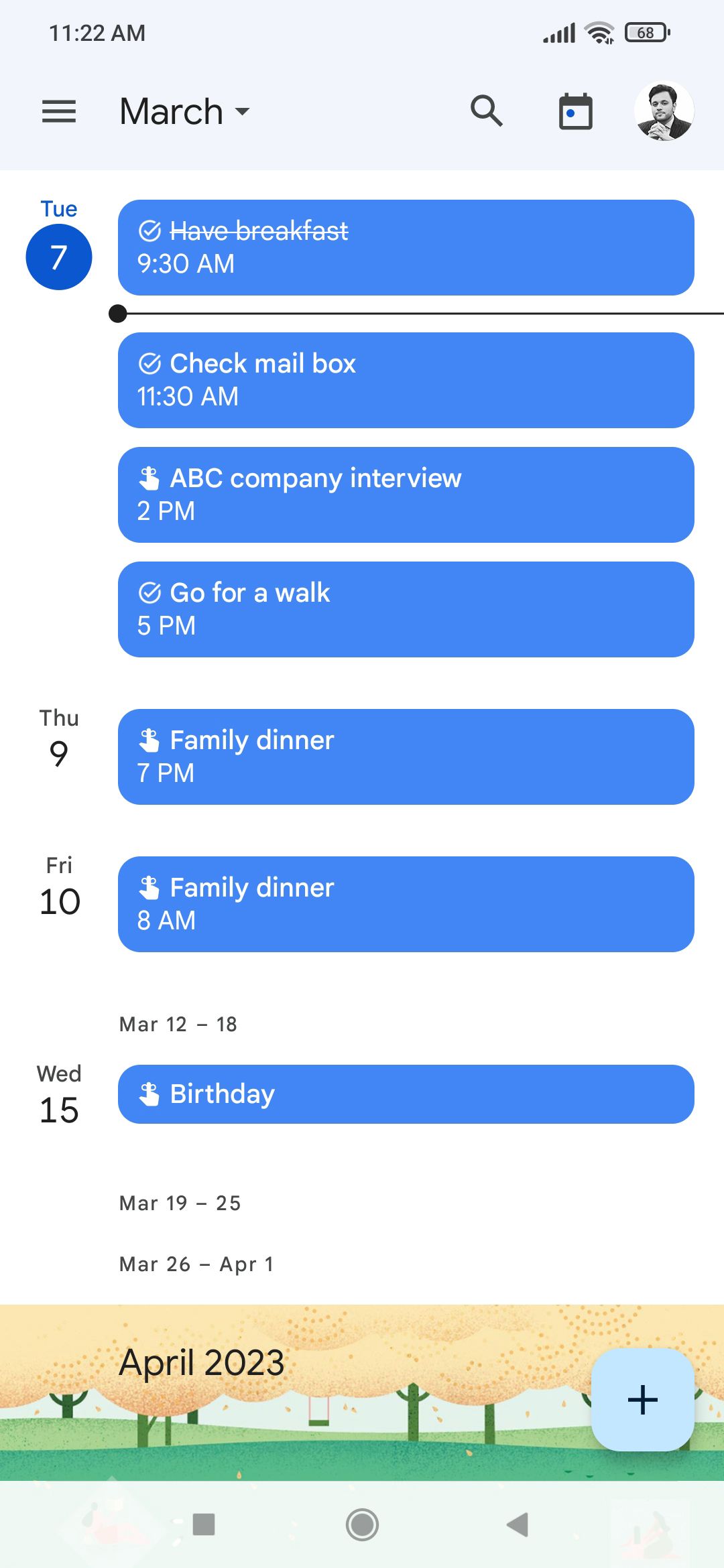The image portrays a detailed to-do list displayed on a mobile phone screen. The background features a light gray rectangle in the top quadrant. The to-do list itself has a white backdrop, with each task presented on navy blue rectangles with rounded edges. These tasks include dates on the left side and primarily black text, with one entry in blue text. 

At the bottom of the screen, the month "April 2023" is prominently displayed. Below this, there's a cartoon-like illustration of a nature park, adding a touch of whimsy. 

The mobile phone's status bar at the top reveals the current time on the left and icons for signal strength, Wi-Fi, and battery on the right. 

Specific entries on the to-do list include:
- Tuesday, the 7th: "Have breakfast at 9:30 AM" (already checked off) and "Check mailbox at 11:30 AM."
- Thursday, the 9th: "Family dinner at 7 PM."
- Friday, the 10th: "Family dinner at 8 PM."
- Wednesday, the 15th: "Birthday."

Overall, the image provides a snapshot of someone's organized schedule on their mobile device, blending functionality with a bit of visual charm.